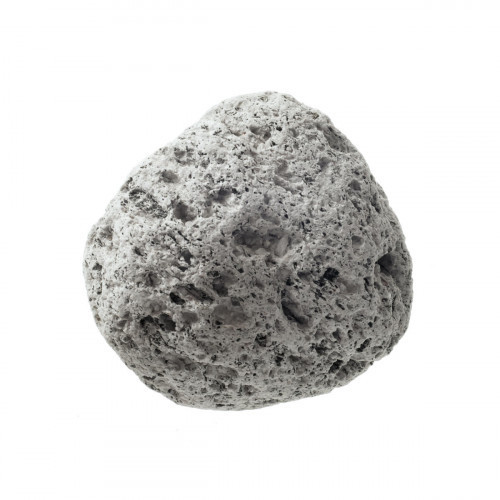This image shows a primarily white rock with a light gray or dirty white hue, featuring numerous darker gray and black holes and specks. The rock is porous, with various crevices, chips, and pores scattered throughout its surface. It's not perfectly round, having an overall conical shape with a gradual point at the top. The rock has a prominent larger hole in the middle and a longish hole towards the bottom of this central hole. Set against a pure white background, the detailed texture and irregular shape of the rock are highlighted, showcasing its potentially moon rock-like appearance.